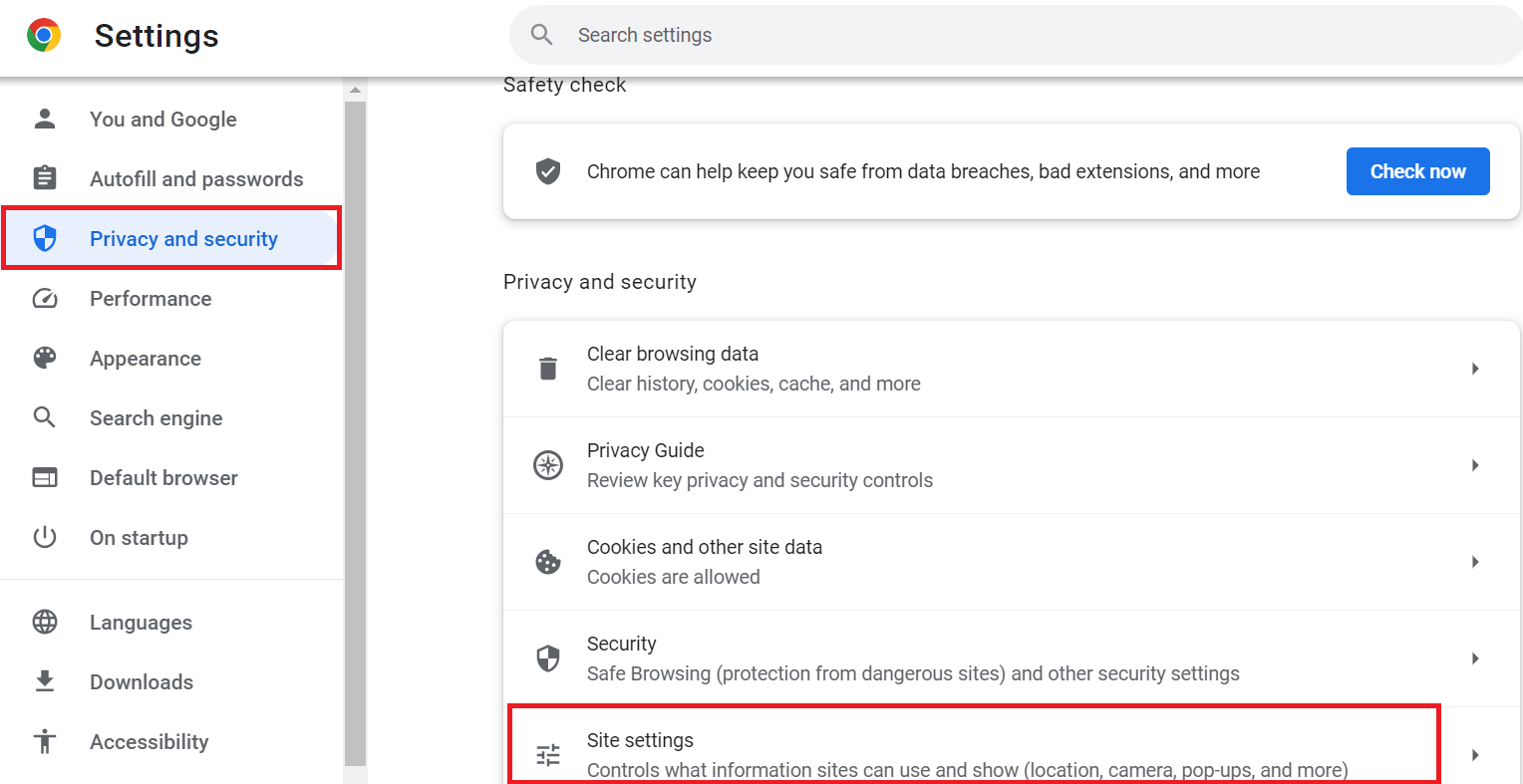A screenshot taken from the Google Chrome browser shows the 'Settings' menu where various user preferences can be configured. The focal point of the image is the 'Safety Check' section, which offers users the option to check if Chrome can protect them from data breaches, harmful extensions, and other security vulnerabilities by clicking a "Check now" button. Below 'Safety Check,' several other settings related to privacy and security are visible, including options to clear browsing data, complete a privacy guide, manage cookies and other site data, configure security measures, and control site settings such as permissions for location, camera access, and pop-ups. Additionally, the left-hand menu displays a comprehensive list of other customizable settings categories, including 'You and Google,' 'Autofill,' 'Passwords,' 'Performance,' 'Appearance,' 'Search Engine,' 'Default Browser,' 'On Startup,' 'Languages,' 'Downloads,' and 'Accessibility.' This detailed interface allows users to finely tune their browsing experience and enhance their online security and privacy.